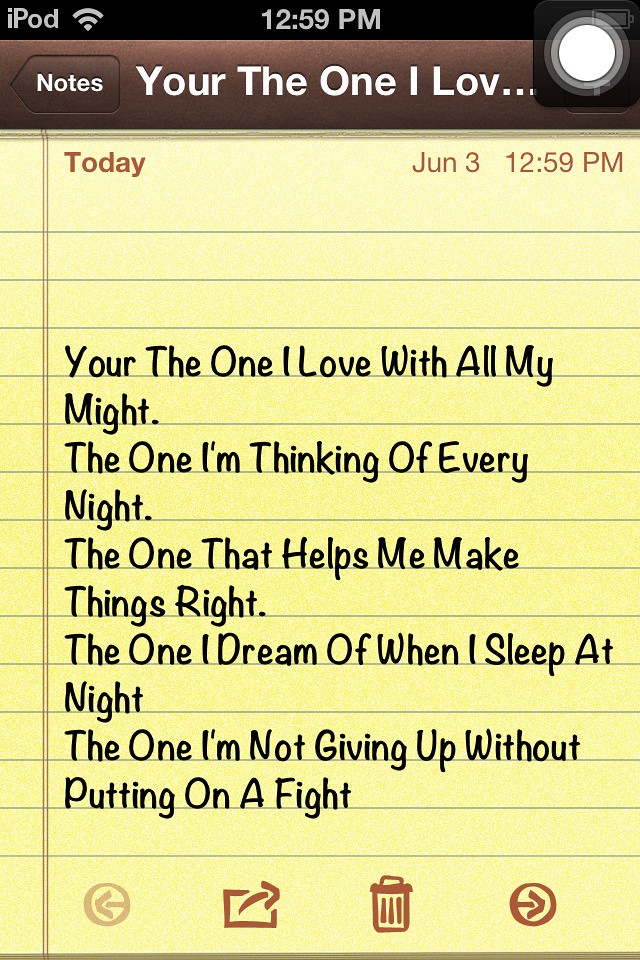This image is a detailed screenshot of a digital notes app on a mobile device, possibly an iPod. At the top, there is a black rectangular strip displaying the time "12:59 p.m." in white font, the word "iPod" on the left, a Wi-Fi symbol, and a small camera lens icon on the right. Below that, a brown rectangular area houses the word "Notes" in white font, and the phrase "You're the one I love..." with "LOVE" partially cut off. The main background resembles a yellow lined notepad.

Centered on the notepad background are the words "Today," "June 3," and "12:59 p.m." in dark brown text, marking the date and time. Below this, in black font, is a heartfelt poem written over several lines:

"You're the one I love with all my might  
The one I'm thinking of every night  
The one that helps me make things right  
The one I dream of when I sleep at night  
The one I'm not giving up without putting on a fight"

Despite a typo where "You're" is misspelled as "Your," the text is clear and expressive. At the bottom of the screen, additional icons appear: a left arrow inside a rectangle, a share icon, a trashcan, and a right arrow, facilitating navigation and actions within the notes app.